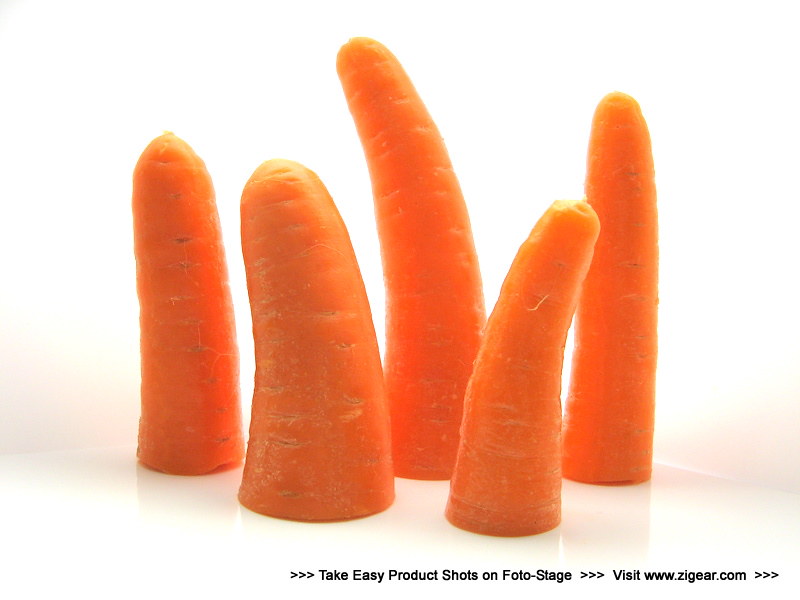This image is a polished advertisement featuring five severed carrot tips standing upright on a glossy white surface, creating an unsettling visual that resembles severed fingers. Each carrot tip is carefully cut and arranged against a stark white background, with some carrots standing straight and others slightly curved. The photo highlights the clean cuts and varying thicknesses of the carrots, emphasizing their rounded, pointy ends. Beneath this peculiar arrangement is a promotional message in black text, punctuated with arrows pointing to the right. It reads, "Take easy product shots on photo stage. Visit www.zygear.com," with "photo stage" styled as "F-O-T-O stage," and the address accompanied by more arrow-like symbols.